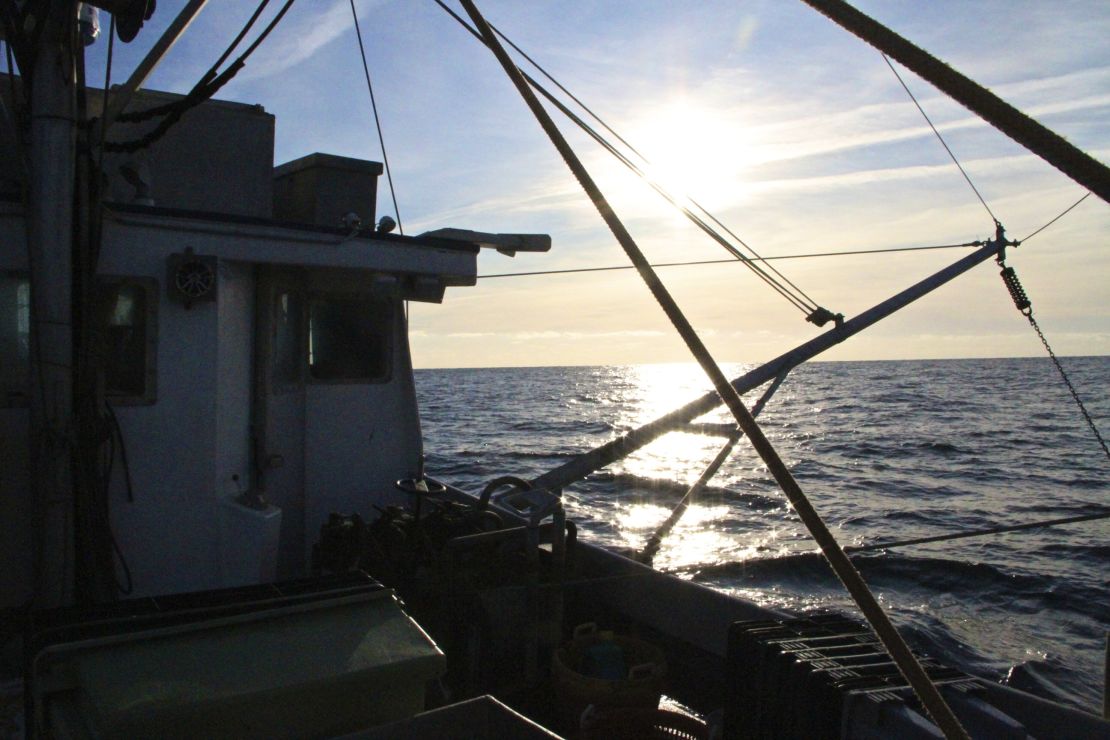The photograph captures a scene from the front of a fishing boat, pointed diagonally towards the back and out to sea. A portion of the white cabin frame of the catamaran is visible on the left side, along with metal pipes and ropes connected to the unseen masts. The snapshot is taken during the late afternoon, with the sun still in the sky and reflecting brightly on the calm, blue ocean waters. The horizon features a blend of light orange and brownish clouds, transitioning into a blue sky with a thin haze of clouds. The overall lighting suggests the approach of dusk, casting a serene and tranquil ambiance over the open sea.